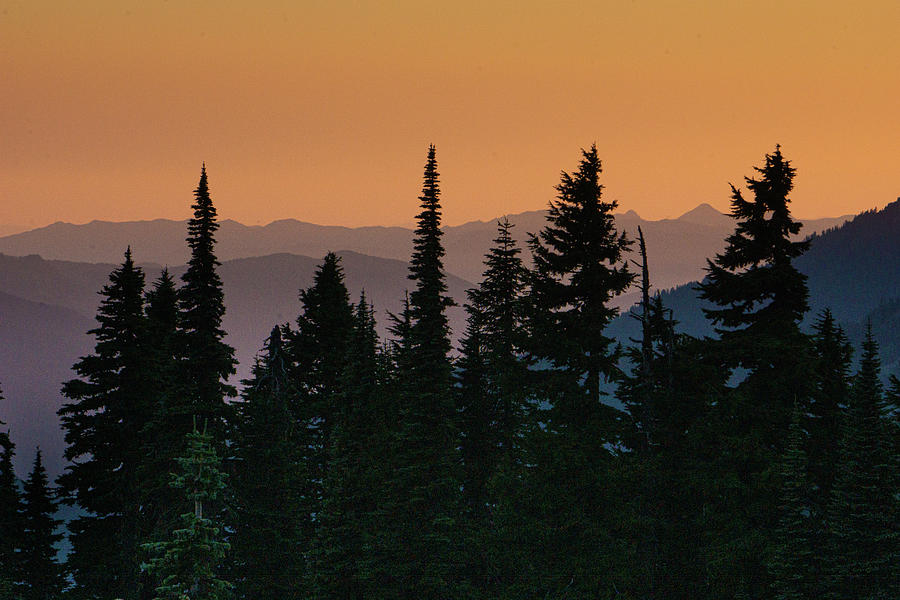A high-angle view capturing the serene beauty of a forested landscape at twilight, either as a photograph or a painting. The foreground is dominated by approximately twelve tall pine trees, their tops showing in varying shades of dark green, some nearly black, suggesting they are cast in shadow. Visible amidst these darker trees is one lighter green tree, adding contrast. The lack of visibility of the trees' bases further anchors the elevated perspective, possibly from a hill, drone, or treetop vantage point. Beyond the forest, an ethereal mountainscape unfolds with four indistinct mountains bathed in muted purplish tones, contributing to the sense of foggy distance and tranquility. Above this, the sky is an enticing gradient of orangey-yellow, transitioning into a soft pinkish hue, indicative of either dawn or dusk. The overall color palette is dusky and subdued, enhancing the enigmatic and tranquil atmosphere of the scene.